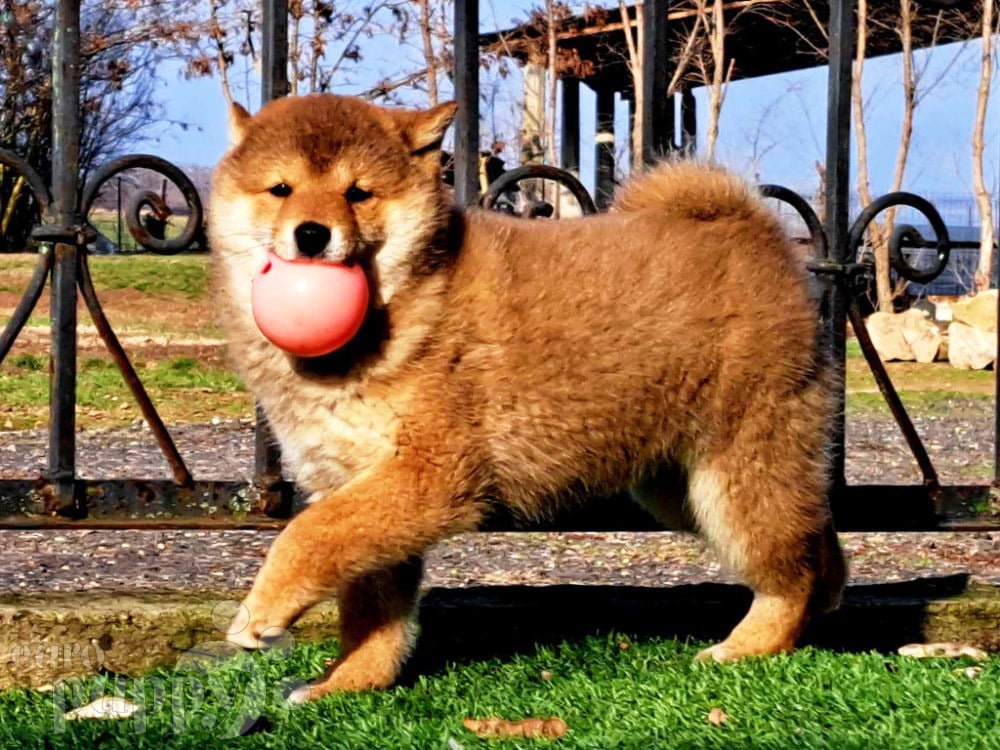The image captures a playful, fluffy chow puppy with a vivid reddish-brown coat and a charming, cream-colored chest. The pup, exuding happiness, is depicted with its left paw slightly raised as it walks on lush green grass in a park setting. Its face, with striking dark black eyes and nose, is turned towards the camera, revealing the pink ball it proudly holds in its mouth. The background features a black wrought iron fence, beyond which are trees, grass, dirt, and a hint of blue sky, enhancing the joyful and lively atmosphere of the scene. The photograph, taken in a realistic style, showcases the puppy's thick fur that transitions from light orange on its chest to darker hues on its head and belly, depicting a moment of pure canine bliss.